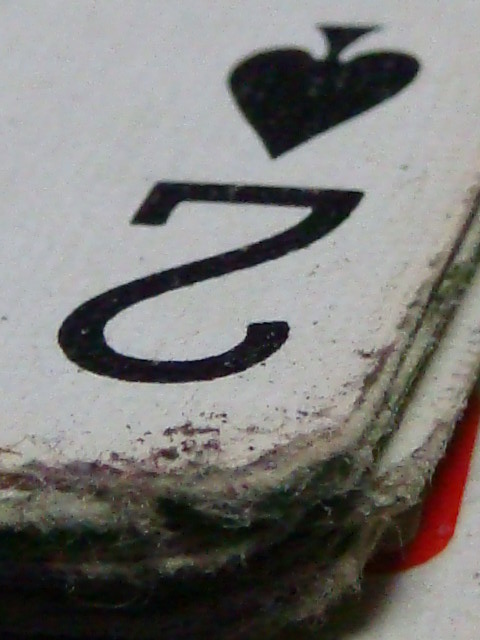This grainy, vintage-style photograph showcases a close-up view of a stack of white playing cards, emphasizing the textured quality associated with older images. Dominating the frame is the prominent two of spades, displayed in sharp black font while partially obscured cards lie beneath. The stack rests atop a white object, offering a subtle glimpse of red peeking through, hinting at a hidden layer or secondary object.

The cards themselves exhibit visible signs of age and neglect, with one corner prominently afflicted by mold in various hues—green, purple, gray, and white—which also trails along the card's side. The white surface of the card has not only suffered from mold but also shows areas where the material has peeled away, revealing the card's deterioration. Additionally, the white object supporting the cards displays minor dotting in one corner, further emphasizing the overall sense of decay present in the image. The photograph is tightly cropped, adding an intimate and concentrated focus on the distressed playing cards and their immediate surroundings, with no extraneous objects included in the frame.